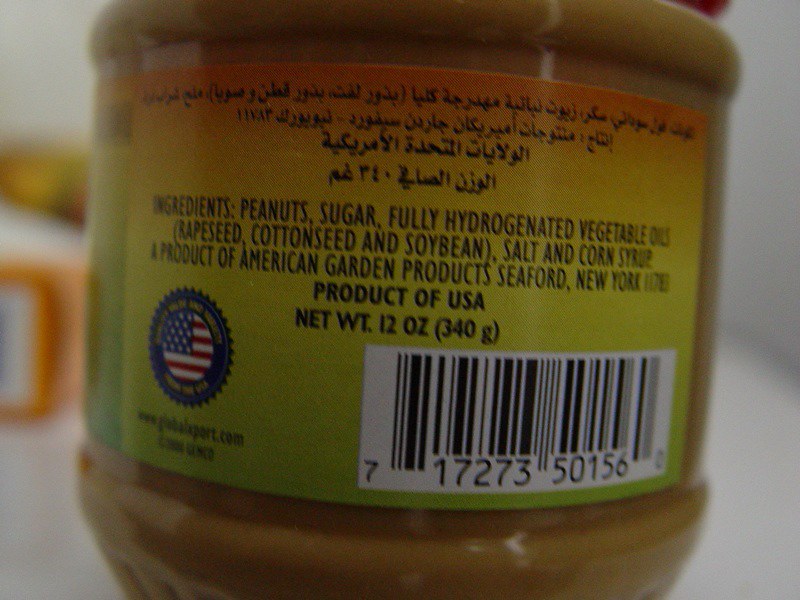The image depicts a wide, plastic jar of peanut butter. The label on the back of the jar features text in what appears to be Arabic, along with the following ingredients listed in black writing: peanuts, sugar, fully hydrogenated vegetable oils (rapeseed, cottonseed, and soybean), salt, and corn syrup. The label also indicates that the product is manufactured by American Garden Products, located in Seaford, New York, USA, with a net weight of 12 ounces. In the left corner of the label, a URL ending in 'port.com' is partially visible. Additionally, there is a barcode at the bottom with the number 71727350156. A small symbol featuring a flag is also present on the label.